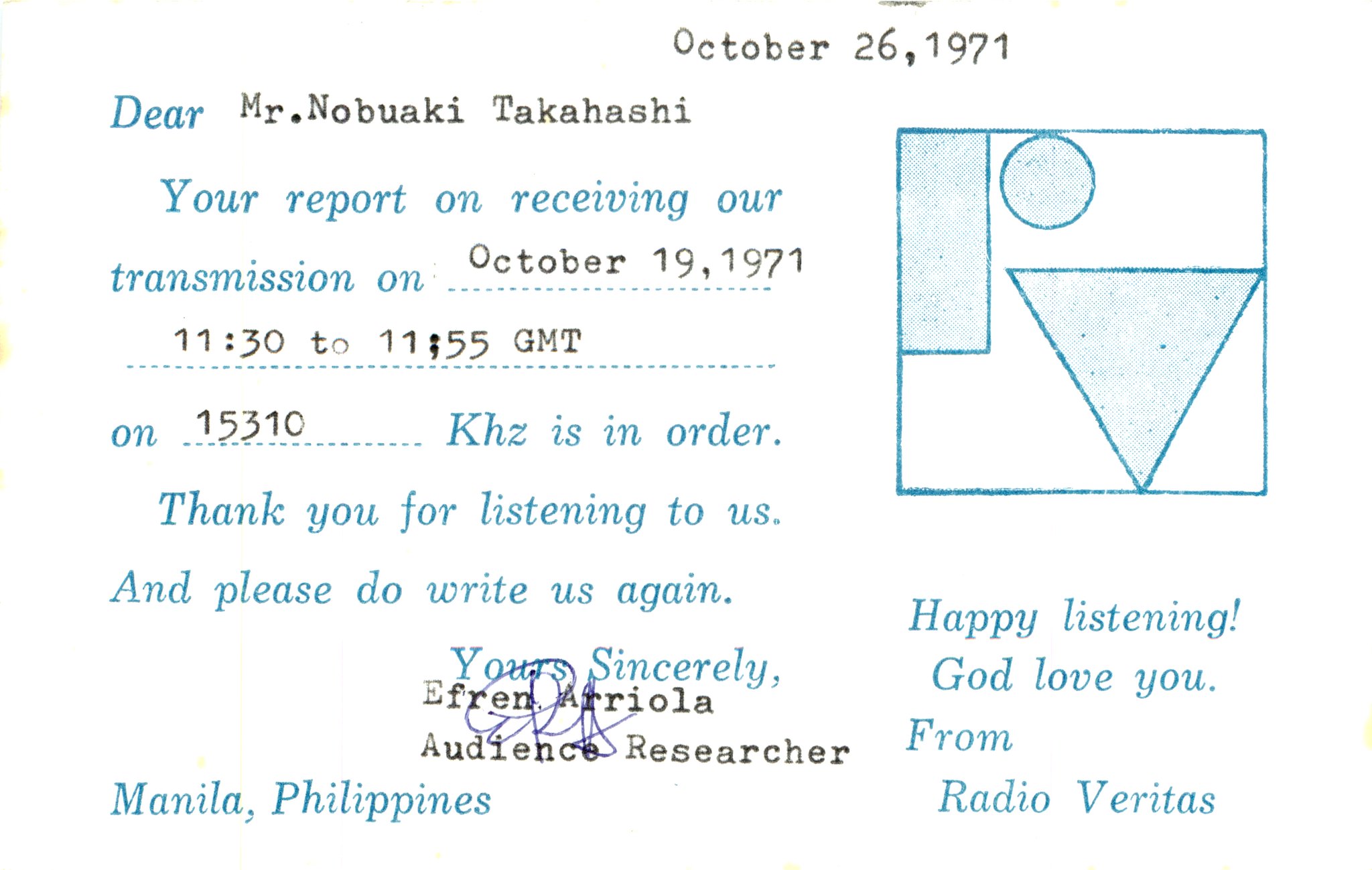This is an image of an old telegram-style letter, dated October 26, 1971, from Radio Veritas in Manila, Philippines. The document consists of a small white piece of paper with pre-printed blue text, and additional details typed in black using a typewriter. At the top, it addresses "Mr. Nobuaki Takahashi" and references a report on receiving a transmission on October 19, 1971, from 1130 to 1155 GMT on 15310 KHZ. The letter reads: "Thank you for listening to us, and please do write us again." It is signed "Yours sincerely," with the typed name "Efren Areola, audience researcher" beneath it. In the lower section, "Manila, Philippines" is printed in blue. In the upper right corner, a blue and white geometric logo featuring a square, rectangle, circle, and triangle appears. Adjacent to the logo, the text "Happy listening, God love you from Radio Veritas" is printed in blue.